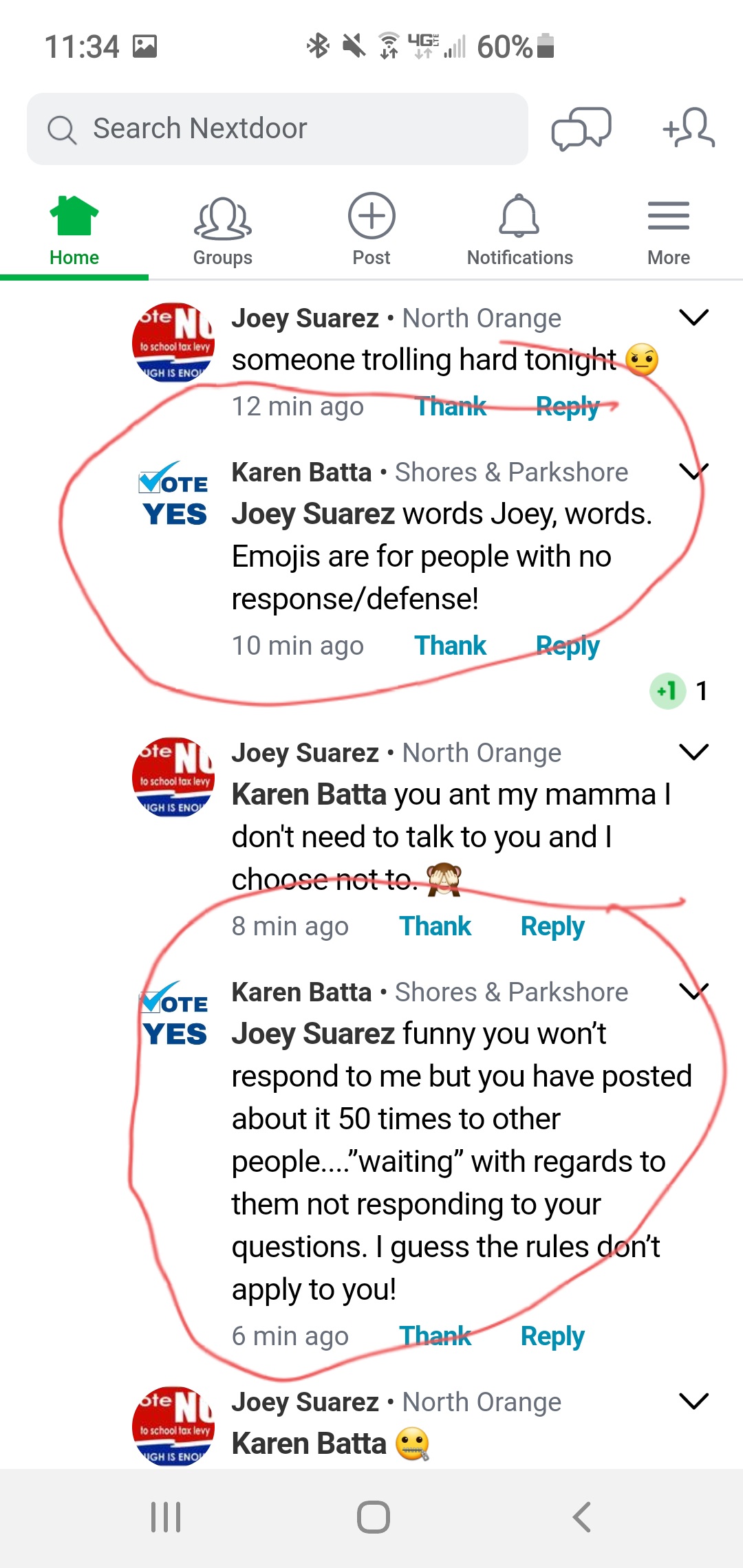This detailed caption describes a screenshot taken from a mobile device. 

At the top of the screen, typical mobile phone icons are visible, including Bluetooth connection, the current time, network connection status, and battery level. The main content of the screenshot displays the interface of a mobile application. At the top of the app interface is a search bar with the placeholder text "Search Next Door." Below the search bar, there is a navigational menu featuring icons for "Home," "Groups," "Add a new post," "Notifications," and an option to access more settings through three vertical grey lines. The "Home" icon is highlighted in green, indicating it has been selected.

The focal point of the screenshot is a list of user comments, which appear to involve a political debate. The users have icons indicating their stances, such as "Vote Yes" and "Vote No." Specifically, two comments from a user named Karen Batter, who uses a "Vote Yes" icon, are prominently marked. These comments are circled with red pen marks, drawing attention to them within the discussion.